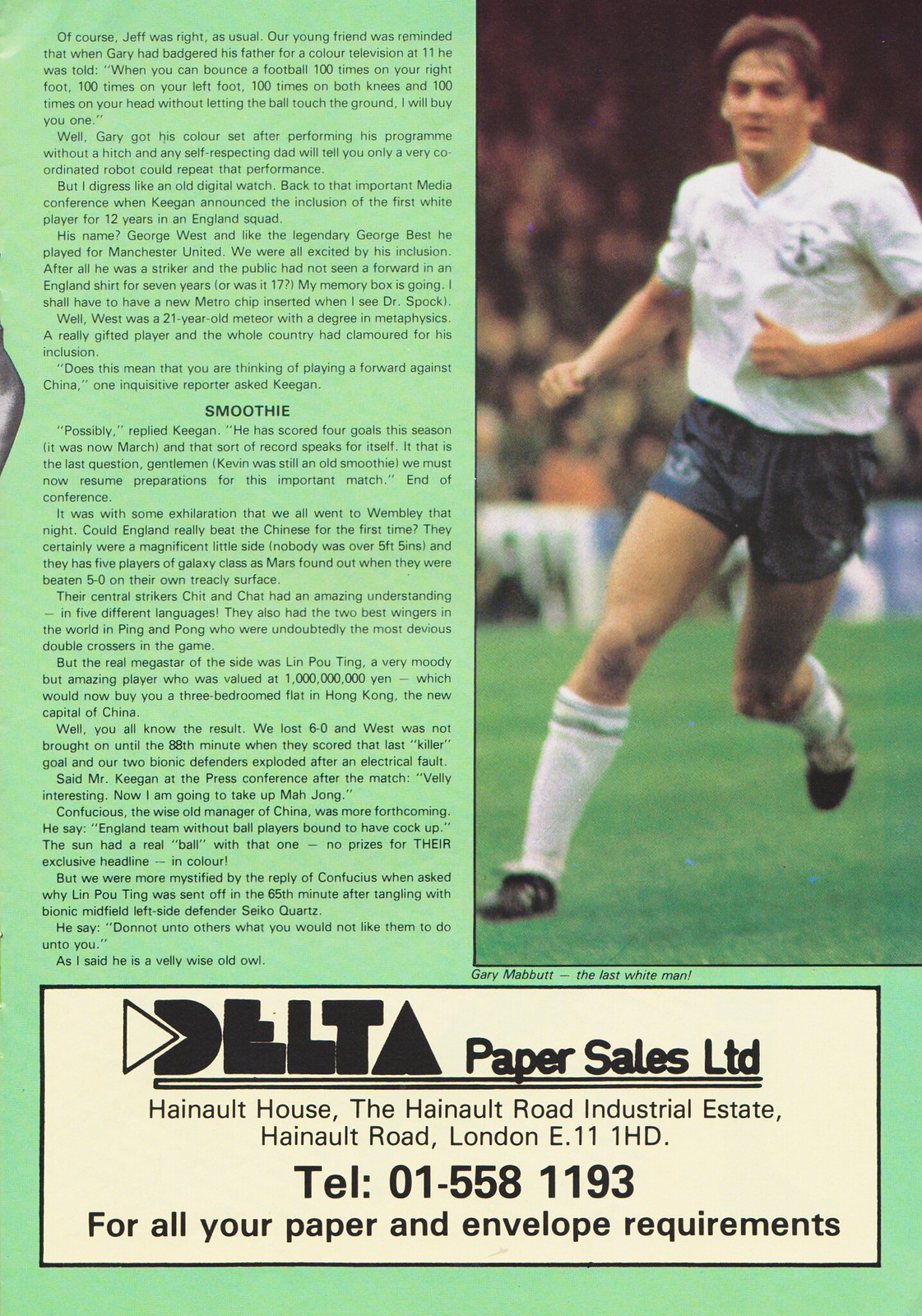The image is a detailed page from a soccer program with a background in key lime green. On the right-hand side, there is a photograph of a man in motion, identified as Gary Mabut, running on a field. He has dark hair and is dressed in a white T-shirt, navy blue shorts, white socks, and black sports shoes. Spectators can be seen in the blurry background. The top half of the left-hand side of the page comprises several paragraphs of text, likely discussing the game Gary Mabut is playing in or providing information about him, with a notable title in dark print that reads "Smoothie." Below the article and photo, there is an advertisement with a tan background for Delta Paper Sales Limited, which includes their address at Honduit House, Honduit Road Industrial Estate, Honduit Road, London, E.111HD, and their phone number, TEL 01-558-1193, along with a tagline, "For all your paper and envelope requirements."